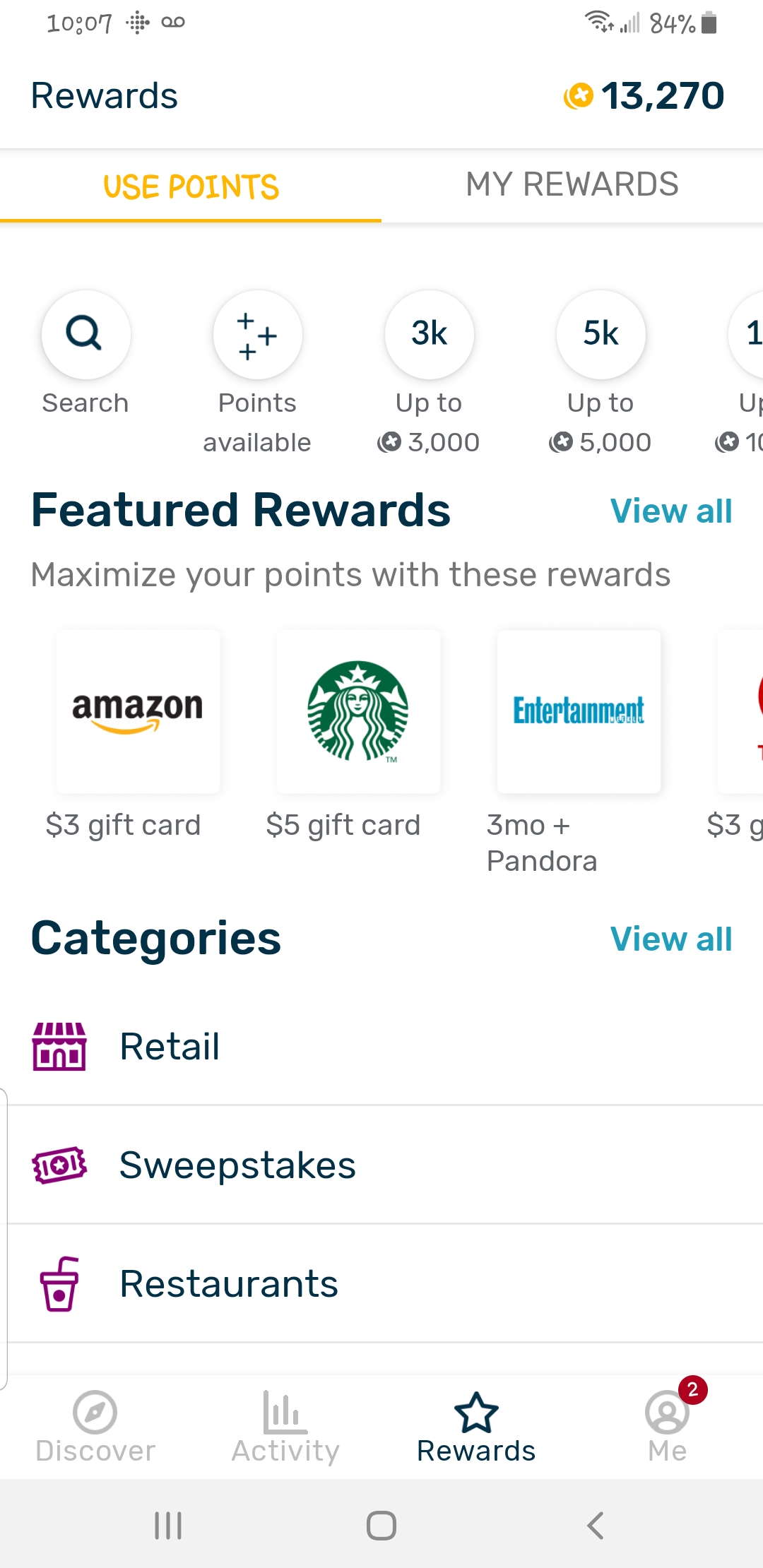The screenshot shows the Fetch Rewards app interface on a smartphone, highlighting various features and reward options available to the user. At the top of the screen, the user's points balance is prominently displayed at 13,270 points. Below this, two main sections are visible: "Use Your Points" and "My Rewards," accompanied by a search function for ease of navigation.

Further down, the app features three circular icons indicating point thresholds with labels: "Points Available," "3K," and "5K," which correspond to rewards that can be redeemed for up to 3,000 and 5,000 points respectively. Following this section, the app showcases "Featured Rewards" with a prompt to "View All" options. Highlighted rewards include a $3 Amazon gift card, a $5 Starbucks gift card, and a 3-month subscription to Entertainment Weekly plus Pandora.

Below the featured rewards, the app categorizes rewards into different sections such as "Retail," "Sweepstakes," and "Restaurants," among others. This section ends with an option to "View All" categories, indicating the possibility to scroll further for more reward options.

At the bottom of the screen, a navigation bar includes icons for "Discover," "Activity," "Rewards," and "Me." The "Me" icon has a red notification badge with the number 2, signaling that the user has two unread notifications.